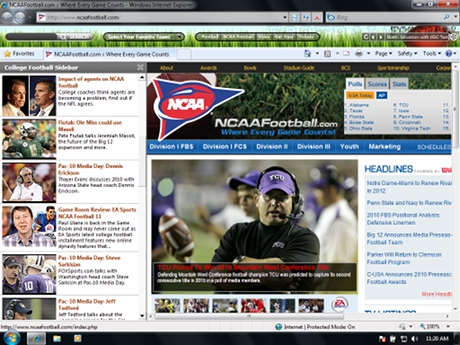Screenshot of an early 2000s NCAA Football webpage displayed in Windows Internet Explorer. The nostalgic interface features several sections and highlights, indicative of older web design. On the left, six sidebar boxes likely showcase college football topics, though the text is blurry and difficult to discern. Headings such as "Impact of Agents on NCAA Football" and incomplete titles referencing Ole Miss hint at typical college football news articles. A prominent image depicts a TCU coach wearing a purple hat and black shirt, though the specific context is unreadable. Adjacent to the photograph are headlines including, "Notre Dame, Miami to Renew Rivalry in 2012," reinforcing the dated nature of the page. Above these sections, navigation tabs are displayed, listing options such as Division 1 FBS, Division 1 FCS, Division 2, Division 3, Youth Marketing, and Schedules. The page captures a busy, content-rich layout from a past era of internet browsing.